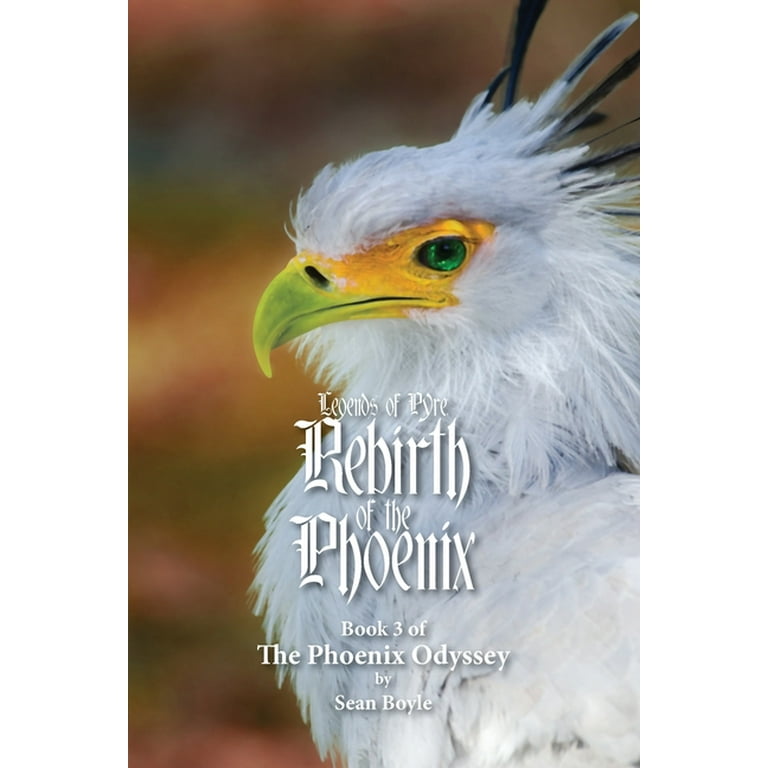The image features the cover of a book titled "Legends of Pyre, Rebirth of the Phoenix, Book 3 of the Phoenix Odyssey" by Sean Boyle. Dominating the cover is a striking illustration of a phoenix with predominantly fluffy white feathers. The tips of the feathers on the top of its head are black, giving it a distinctive appearance. The bird's golden and orange beak is hooked at the tip which is a greenish-yellow color. Its emerald green eye with a dark pupil adds a fierce and serious expression to its demeanor. The soft-focus background blends shades of brown, dark blue, and green, creating a contrast that makes the phoenix stand out prominently. The title is displayed in fancy white lettering, extending from the bird's neck down to its chest. There is also a slight green tinge to the feathers on the phoenix's breast, enhancing the overall mystical and legendary theme of the cover.